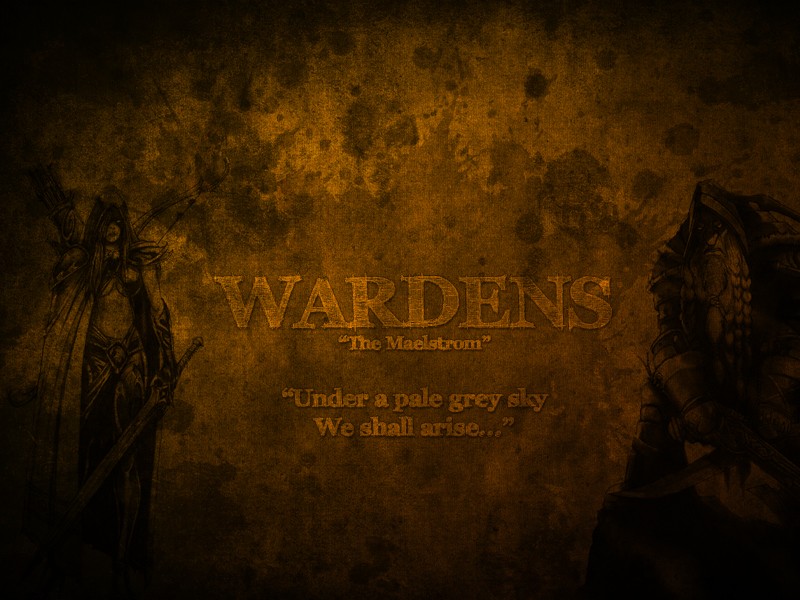The image features a predominantly copper-colored background that is darkly stained, resembling an old piece of cloth. In the center, large capitalized golden text reads "WARDENS," with "the Maelstrom" and "Under a pale gray sky, we shall arise..." in quotes, spanning two lines. On the left, there is a detailed illustration of a female warrior with long, straight hair shrouding her face in shadows. She sports a sleek, superhero-like outfit with her midriff exposed, a flowing cape, shoulder pads, and holds a broadsword in her left hand. Her outfit also includes thigh coverings and possibly a mask, and a bow is visible on her back. To the right of the text stands a brooding male figure with a hood and a long white beard, giving off a wizard-like aura. He wears a gauntlet on his right hand and appears to be holding a battle axe. Both characters are depicted in black lines against the eerie, stained copper background, framing the text in the middle of the image.